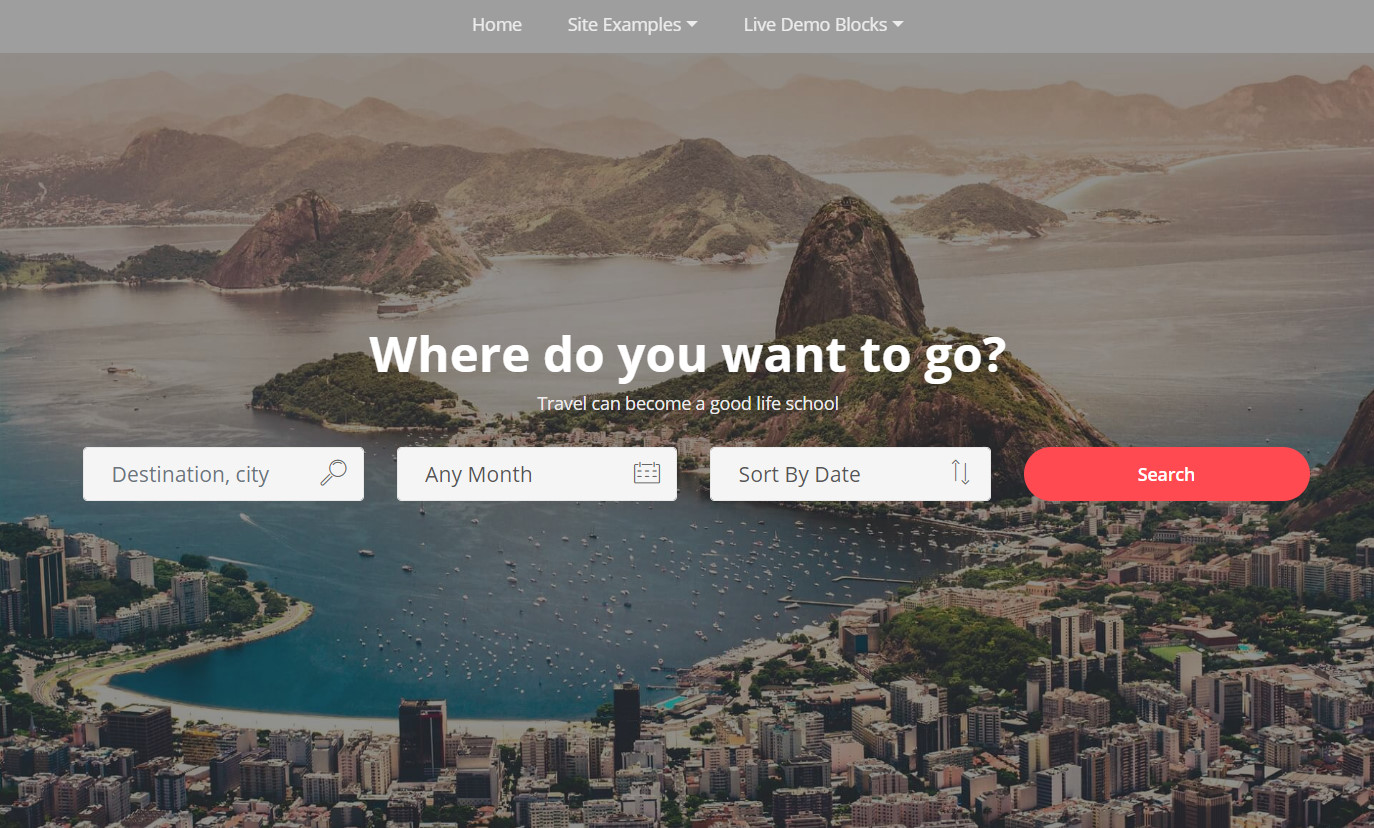The webpage header includes navigation links such as "Home," "Side Examples," "Live Demo," and features a gray sidebar. The main image prominently showcases a picturesque landscape of towering mountains and serene lakes interspersed with lush forests and scattered islands. The backdrop has a misty quality, adding an ethereal touch to the scene. In the center of the image, there is white text asking "Where do you want to go?" accompanied by options for selecting a destination, city, and travel period. A magnifying glass icon and a red oval "Search" button are also present.

Below this search interface, the calendar can be sorted by date using up and down arrows. Off in the distance, tightly packed buildings line the beaches, with boats scattered across the vivid blue waters, hinting at a bustling coastal community potentially in the Caribbean. The lush greenery, vivid waters, and densely populated shoreline evoke a sense of a tropical yet urban escape, possibly mimicking an Airbnb template for travelers seeking an idyllic getaway.